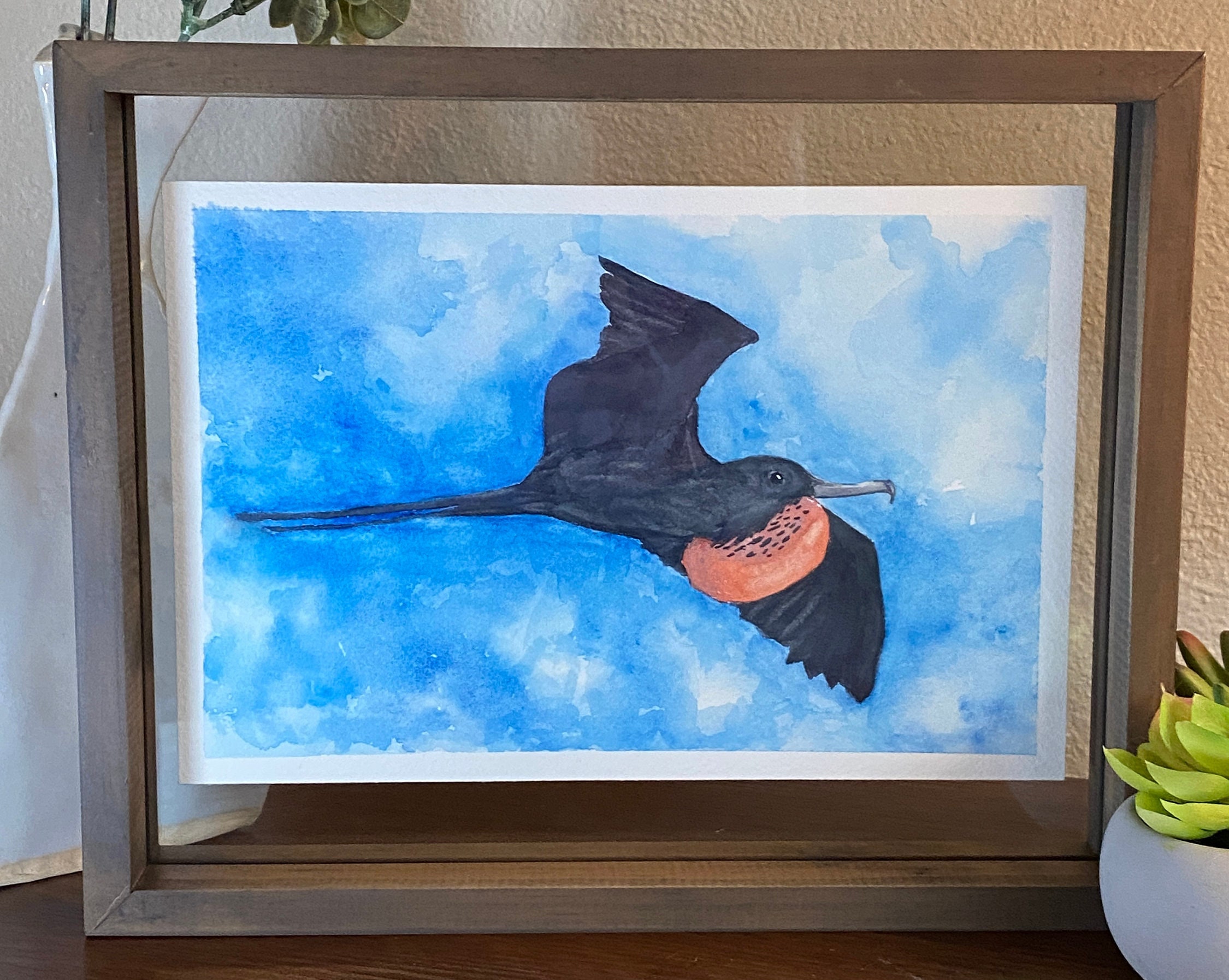In this scene, set against a light brown wall, a brown table serves as the base for an array of carefully arranged items. A very tall, pale blue flower vase can be seen in the background, housing a few leaves and stems that add a touch of greenery to the setting. In front of it, a smaller, round vase holds a delicate green flower, offering a simple yet elegant contrast. A brown wooden picture frame with clear glass stands nearby, showcasing a piece of art. Inside the frame, a white paper backdrop highlights an image of a black bird soaring against a blue sky. The sky is depicted in varying shades of blue with hints of white, emphasizing the bird’s long, thin black tail, expansive wings, striking orange breast, and distinctive long white beak. The overall composition creates a harmonious blend of natural elements and thoughtful design.